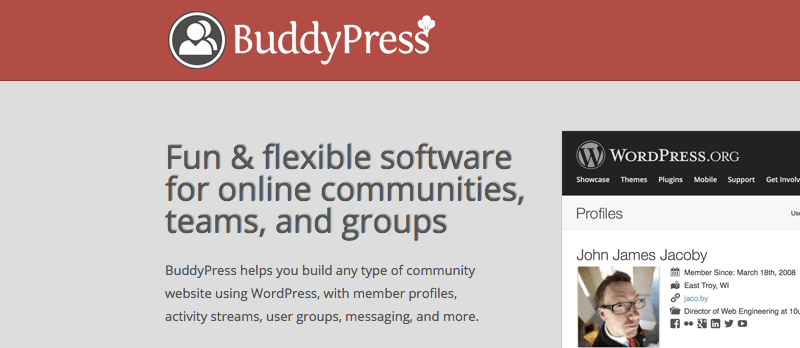The image features a structured layout designed to showcase BuddyPress, a WordPress plugin for creating online communities. At the top of the image is a prominent red box containing a circular logo with two small figures, labeled "BuddyPress." Above the "S" in BuddyPress, three small white balloons are visible. Below this, a large blue box displays the text: "Fun and flexible software for online communities, teams, and groups. BuddyPress helps you build any type of community website using WordPress with member profiles, activity streams, user groups, messaging, and more."

On the right side of the image is a black box featuring a gray box with a "W" inside, representing WordPress.org. This section contains links labeled "Showcase," "Themes," "Pages," "Mobile," and "Support." Adjacent to this is a white box showcasing a user profile for "John James Jacoby," including a small square with his photo and his member details. Several small social media icons, including one for Facebook, are displayed below his information.